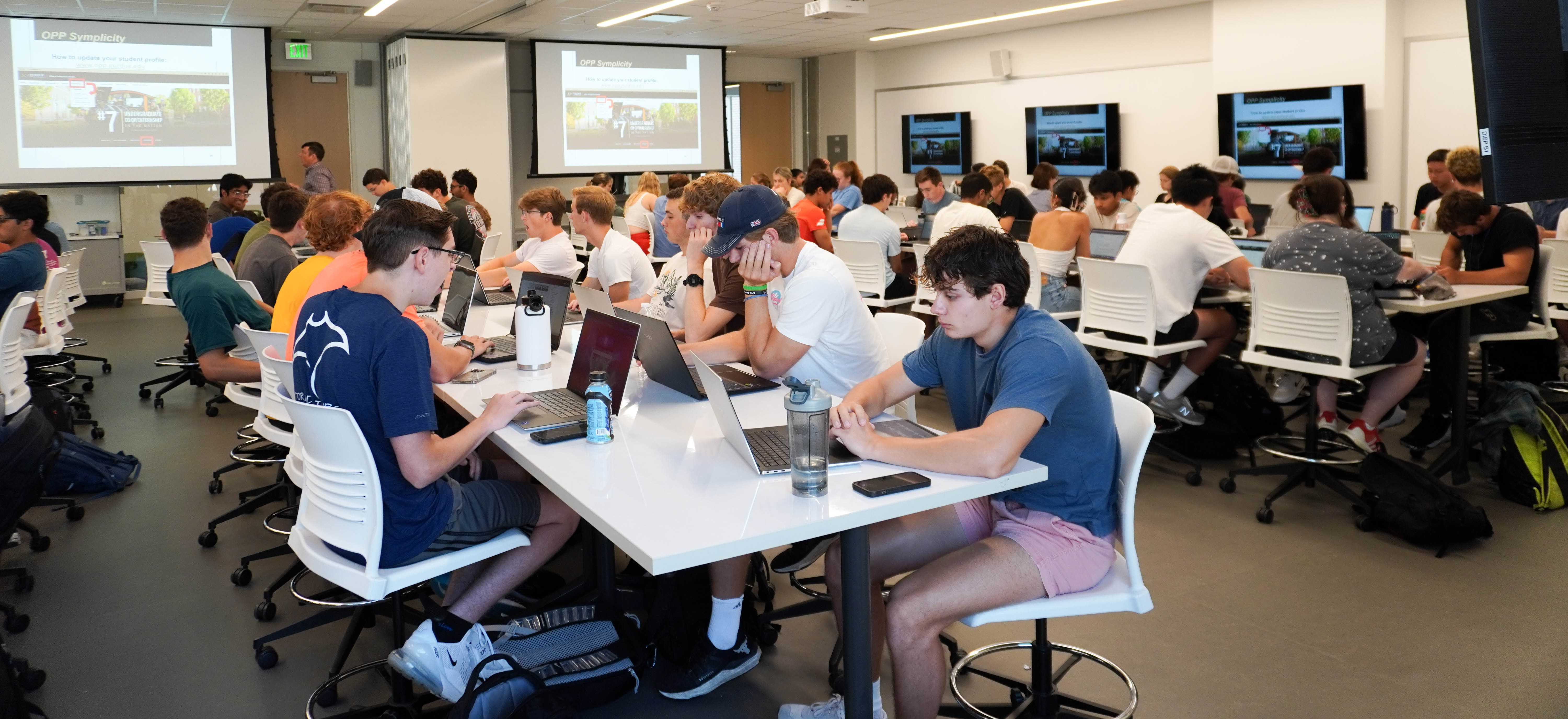This indoor photograph captures what appears to be a bright, modern classroom or a collaborative workspace with a start-up ambiance, specifically oriented toward a tech-savvy, college-aged crowd. The room is populated by numerous young men, casually dressed, seated in white swivel chairs on either side of long, white rectangular tables. Each individual is absorbed in their laptop screens, some with water bottles and phones also on the tables. 

The setting includes multiple rows of tables, with about three tables visible in the image. Although the table on the left is partially out of frame, the people seated there are still visible. In the background, there are a couple of large screens prominently displaying a presentation with the headline "OPP Simplicity," though the detailed content is too blurry to decipher. Additional smaller screens mirror this projection on three other rows, and there's another screen partially visible in the top right corner, facing away from the viewer.

On the right side of the room, a man, likely the presenter, walks towards the left, emphasizing the interactive, lecture-like atmosphere. The room's interior features white walls, brown doors, and grey flooring which adds to the contemporary, minimalist aesthetic of the space.